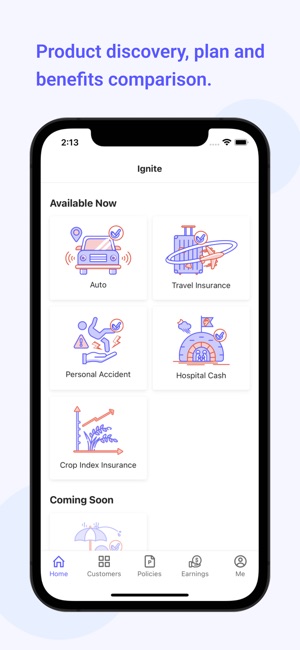In the image, the prominent title "Product Discovery Plan and Benefits Comparison" is displayed in purple text at the top center. Below the title, a smartphone is featured, encased in a black protective cover. The phone's screen showcases an app with the heading "Ignite" positioned prominently at the top. The status bar of the phone indicates a full battery and a strong Wi-Fi connection, with the time displayed as 2:13 in the top left corner.

Beneath the heading "Available Now," the app presents five distinct categories, each enclosed in a square box. In the top left box, labeled "Auto," there's an image of a car driving toward the viewer. To the right, under "Travel Insurance," an airplane is depicted flying in a circular motion. 

The second row includes the category "Personal Accident" on the left, illustrated with a hand helping a person who appears to be slipping. To its right lies "Hospital Cash," symbolized with an igloo icon. The final box, labeled "Crop Index Insurance," features an image of crops growing upwards, completing the array of available insurance options displayed on the app.